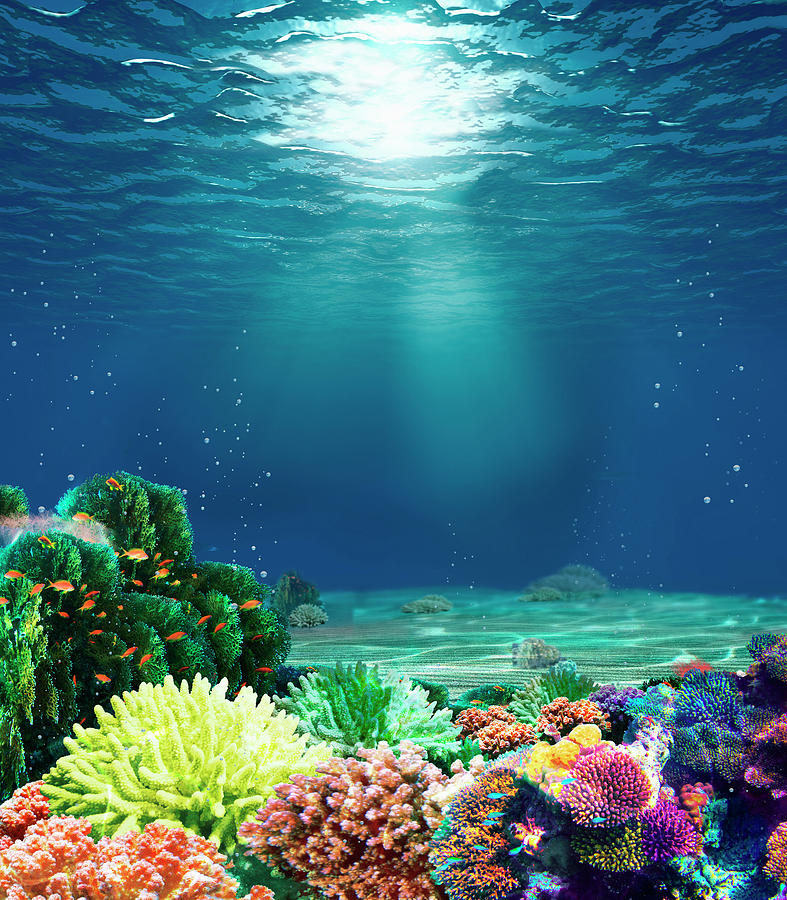This vertical image, possibly a digitally enhanced or created scene, showcases an underwater coral reef bathed in daylight. The water is exceptionally blue and transparent, with reflections of the ocean's surface rippling above. Sunlight penetrates from the top center, casting a radiant glow onto the vibrant coral reefs below. These reefs are a kaleidoscope of colors, featuring green, pink, purple, blue, and reddish hues, and are dotted with various marine animals, including anemones. Small orange fish swim among the corals, adding life to the scene. Air bubbles rise from the sandy ocean floor, further enhancing the vivid and dynamic nature of this underwater vista.